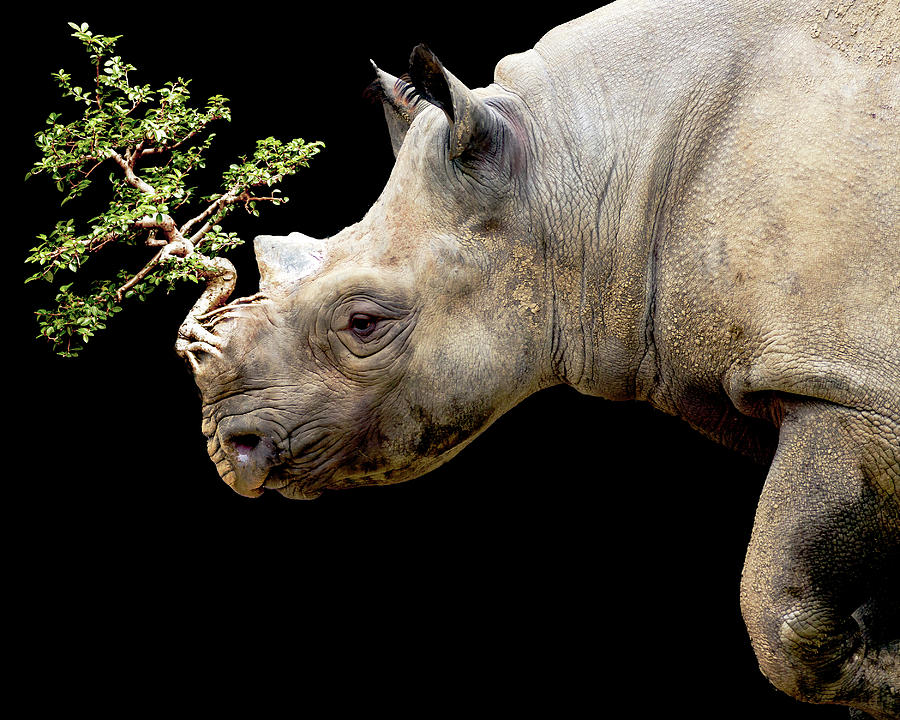The image showcases a highly detailed, photorealistic portrayal of a rhinoceros set against a pitch-black background. The rhinoceros, primarily depicted from a side profile, is facing left, revealing its wrinkled, grayish-brown skin with patches of dirt enhancing its textured appearance. The rhino's eye is open, and its ears, slightly furred, are visible, both positioned forward. Notably, the front horn of the rhinoceros has been digitally replaced with a small, detailed bonsai tree. This tree, rooted in the rhino's nose, features a light brown, spirally warped trunk and branches adorned with small, shiny green leaves. Only the rhino's head, shoulder, and partially bent front left leg are visible, suggesting a forward-leaning stance or a step mid-motion. The overall image blends realism with surrealism, making it evident that the tree substitution is a product of AI or digital editing.